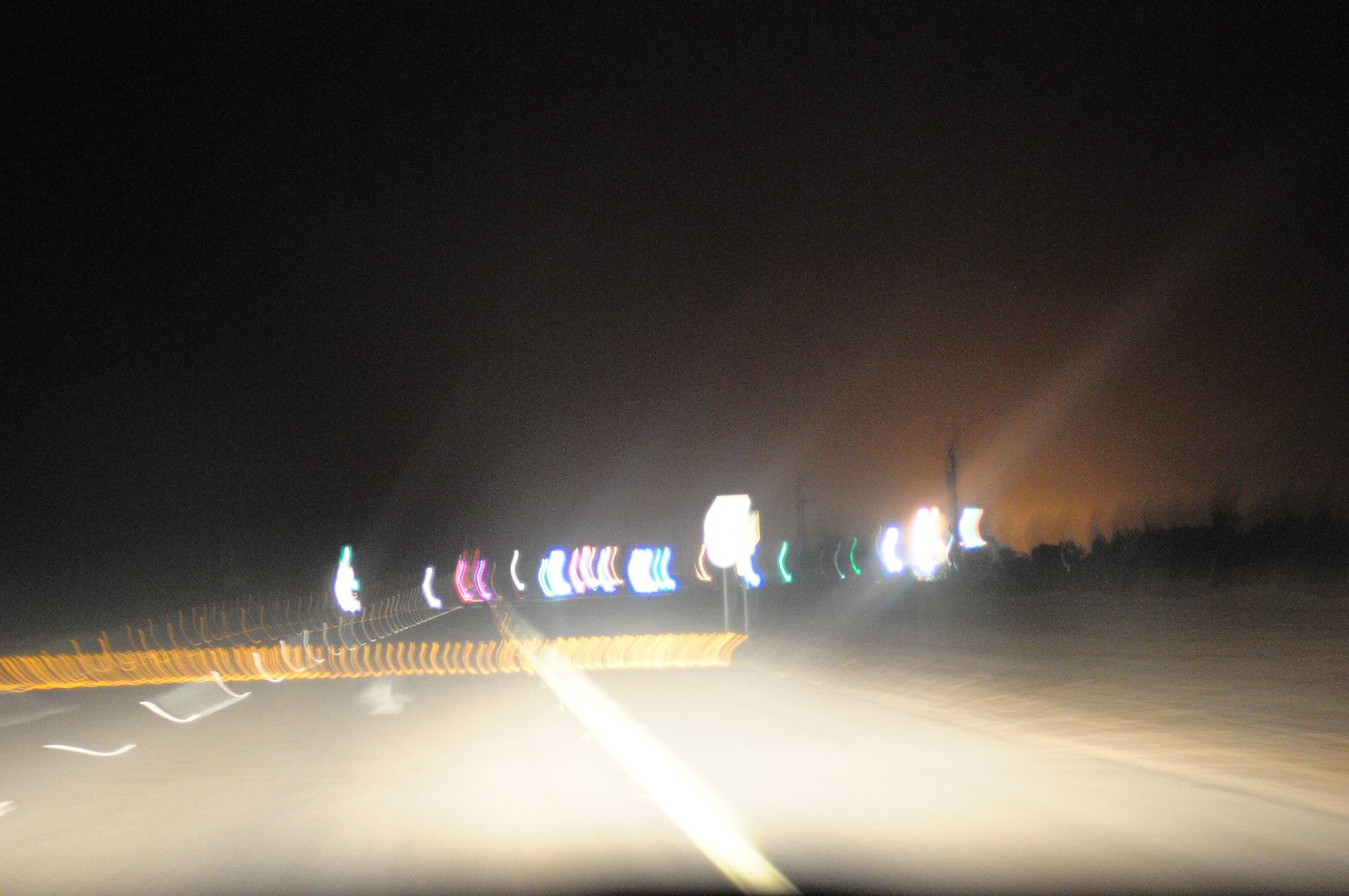This is a color photograph depicting a blurry, night-time roadside scene. The dark sky dominates the top portion of the image, creating a somber background. Near the center, faint orange light slightly illuminates several poles, providing a hint of structure amidst the obscurity. The middle section features a line of variously colored, blurred lights—white, pink, blue, and green—along with larger, lower white lights, which are likely from vehicles on the road or possibly distant buildings.

The roadside, visible at the bottom of the photograph, has a pronounced, wide appearance, distinguished by a thin solid white line running through its middle and another broken white line to the left. Additionally, a mysterious, horizontally stretched out yellow light appears coiled, possibly indicating a moving object whose shadow remains indiscernible. Towards the right side, an area that seems to depart from the road might be ground, possibly adorned with trees near the horizon. A tall pole stands near the center-right, adding to the array of indistinct forms in this night-time roadside scene.